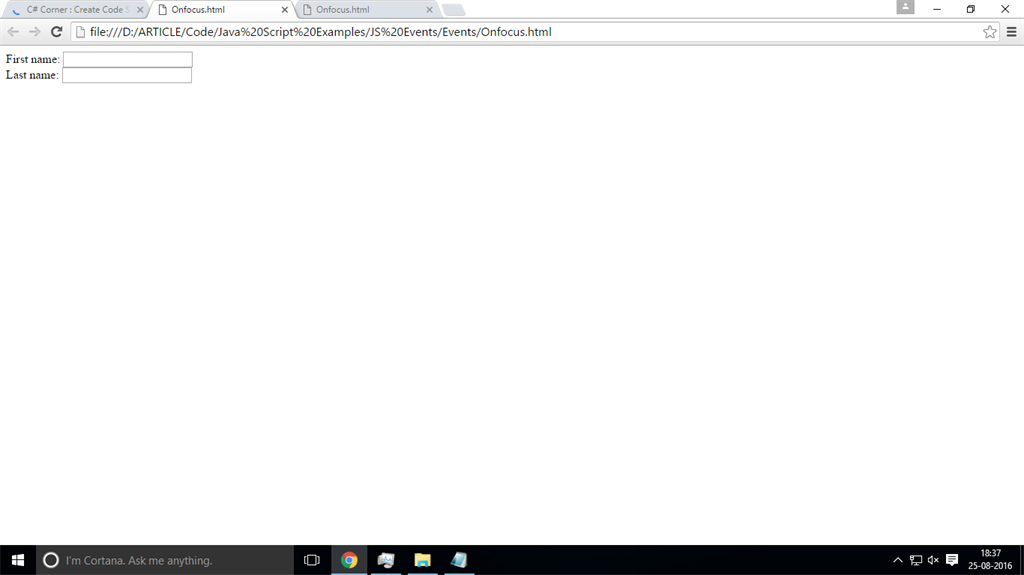**Detailed Caption:**

This image appears to be a screenshot taken from a Windows operating system. The main content is likely displayed within a web browser interface, which is confirmed by standard navigation buttons such as reload and forward arrows. The URL shown in the address bar reads: `file:///D:/article/code/Java%20S%20examples/JS%20events/events/on-focus.html`.

At the top of the browser, multiple tabs are visible. The currently selected tab is titled "on-focus HTML," with an identical tab open to its right. To the far right within the same row are typical browser window buttons: minimize, maximize, and close.

Just below the address bar, two text input fields labeled "First Name" and "Last Name" can be seen, both of which are currently empty. The rest of the web page seems to be blank.

In the browser toolbar on the top right, there's a hamburger menu icon, commonly used for additional options, and a star icon, possibly indicating bookmarking options.

The taskbar situated at the bottom left of the screenshot displays a black square with a white Windows icon alongside a circular "Cortana, Ask me anything" search bar. Nearby are various app icons such as Google Chrome, File Explorer, Settings, and Notepad.

To the bottom right of the taskbar, standard Windows icons are visible, including the system clock showing "16:37," the date "25/08/2016," a speech bubble icon likely for notifications, and other system status icons for network connectivity and sound settings, with the latter appearing to be either muted or set to a very low volume. A power icon is also discernible, indicating options for system power management.

Overall, the page itself is nearly devoid of content, except for the mentioned fields and navigational elements.